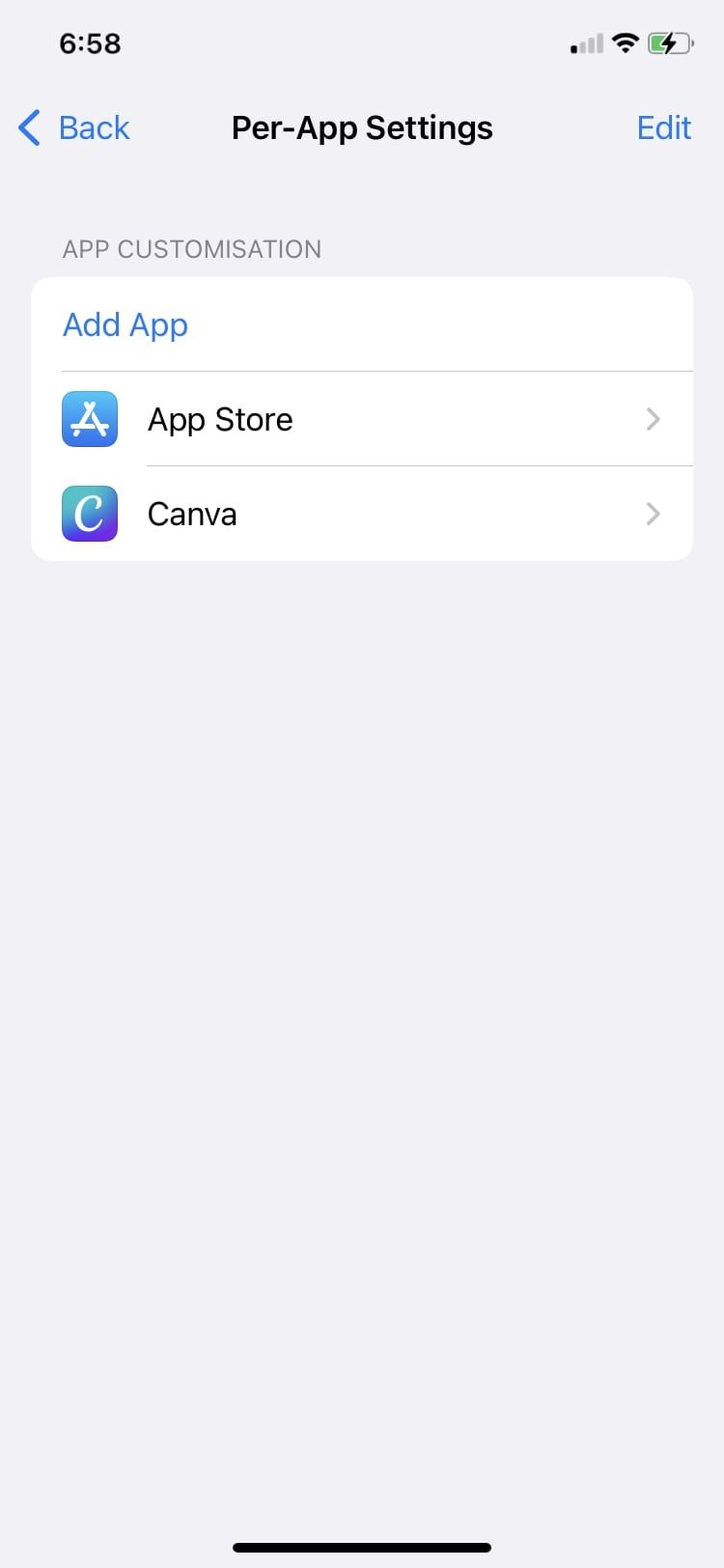This image captures a screenshot from a mobile device, displaying a settings page. At the top of the screen, the title "Per App Settings" is centered between a back arrow on the left and an edit option on the right. Directly below the title is the "App Customization" category, under which an "Add App" button is positioned. Presently, only two apps are listed under this category: "App Store" and "Canva," each accompanied by a right-arrow indicating additional details can be accessed upon tapping.

The lower 70% of the page remains blank, with no further content. At the very top of the screen, the current time is shown as 6:58 AM in the upper left corner. In the upper right corner, three icons are displayed: a cellular signal icon showing one out of four bars, a Wi-Fi icon fully lit with four bars, and a battery icon that is partially filled and displays a charging status without showing a specific percentage.

The minimalistic design and ample unused space suggest a streamlined and uncluttered user interface.